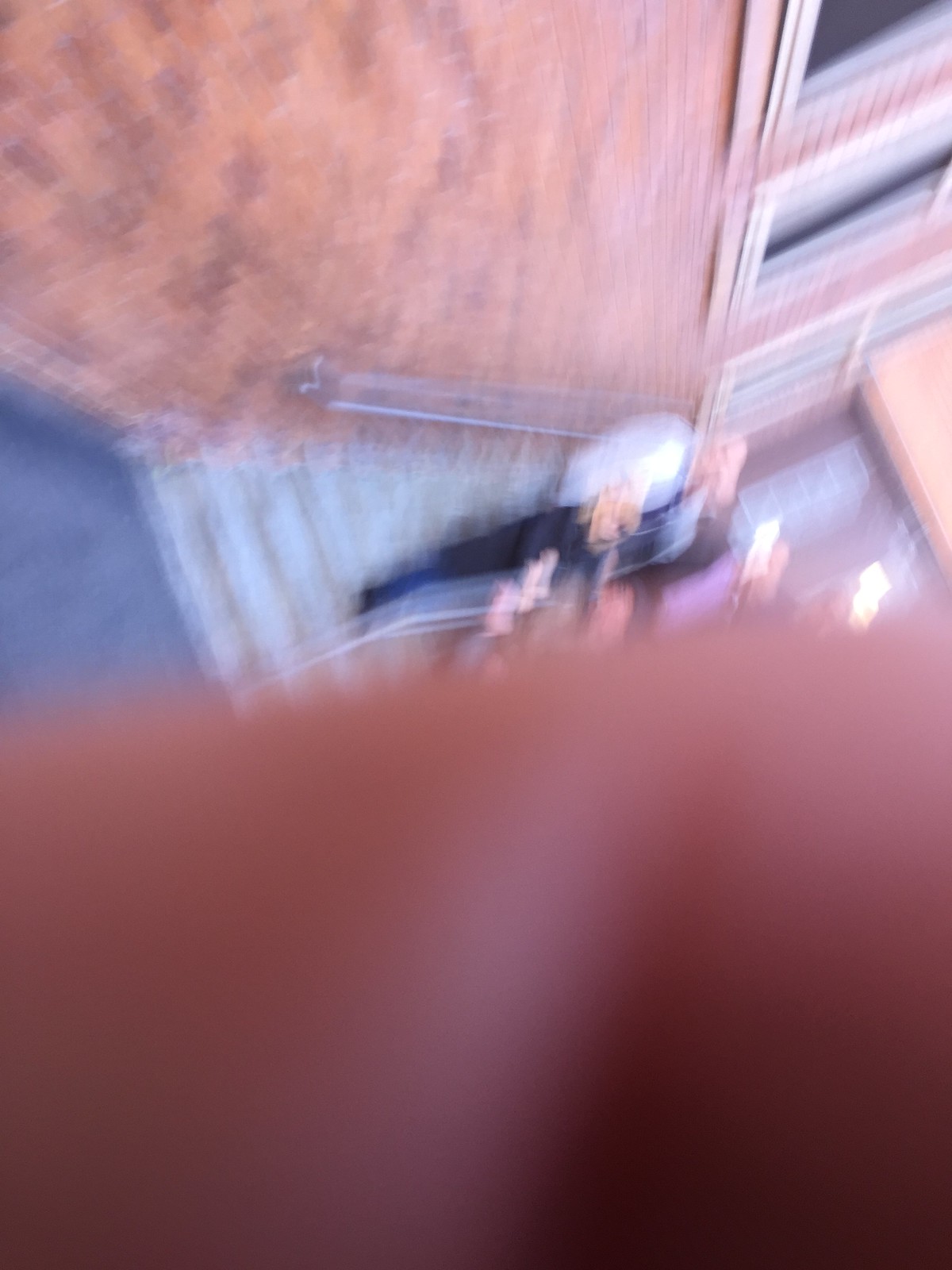This photograph, although blurry, appears to have been taken from a balcony on an upper floor of a building. The vantage point overlooks a set of gray cement stairs, which feature a metal railing on one side and a long metal pole attached to the adjacent brick building on the other side. In the foreground, part of the lens is obscured by the pinkish flesh of someone's finger. On the steps, a bald white man wearing a dark shirt is facing the brick building, while a blonde woman is seen looking in the opposite direction, down the stairs. The composition hints at a candid, urban moment captured amidst the everyday movement of people.